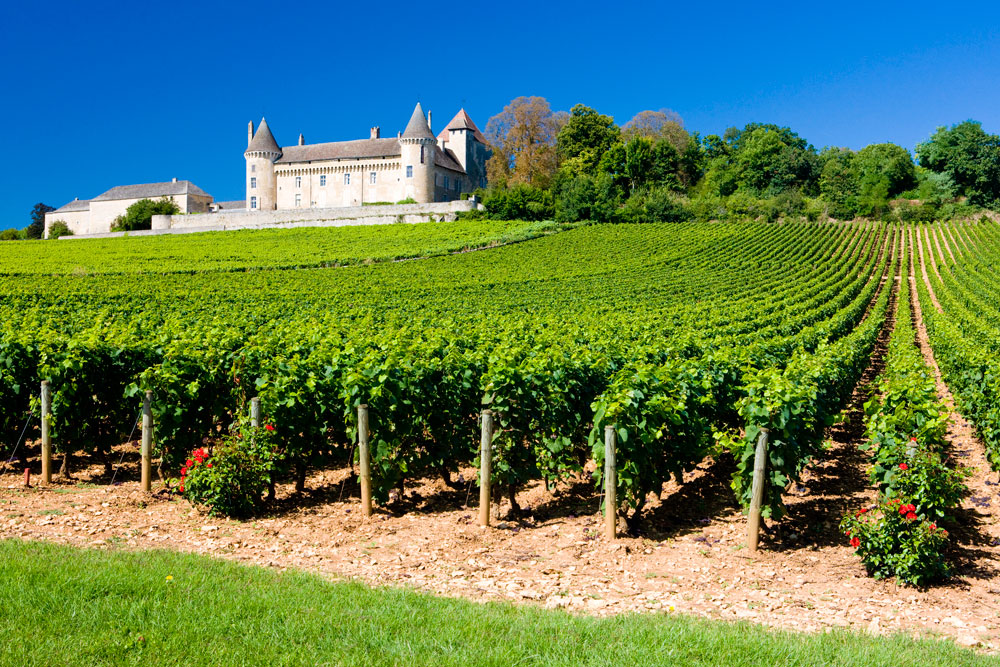This outdoor photograph captures a scenic vineyard under a dark blue sky, with verdant rows of grapevines stretching regally from the left-hand side all the way to the right. The grapevines, interspersed with light-colored brown dirt and occasional plants bearing red flowers, create a vivid tapestry of green and red. In the extreme foreground, a patch of lush green grass frames the scene.

Dominating the upper left corner of the image is a stately stone building that resembles a castle, complete with a dark gray slate roof and at least three to four towers adorning its edges. A stout, gray stone wall encloses the building, adding to its fortress-like appearance. Adjacent to it stands a smaller, similarly colored structure that might serve as additional quarters or possibly stables.

The right side of the background is marked by a tree line, with trees displaying a mix of dark green and a hint of brown foliage, suggesting an early turn toward autumn. The juxtaposition of these lush, full-leafed trees against the brilliant blue, cloudless sky enhances the vibrant and serene atmosphere of the vineyard.